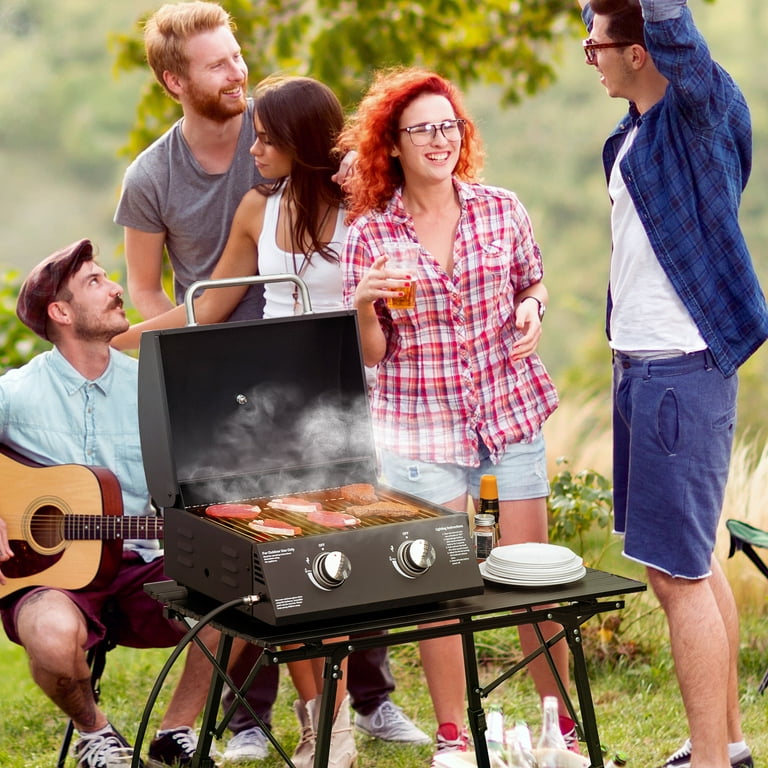In this vibrant outdoor scene, five people are gathered for a barbecue on a sunny day in a grassy area. Centered is a man seated behind a black grill with large silver knobs, playing a guitar and wearing a blue shirt. The grill, situated on a small black table, is cooking six pieces of meat, with a couple of cuts appearing more cooked than the others, alongside a stack of white plates and seasoning items. Behind the seated guitarist stands a man in a gray short-sleeved t-shirt with reddish hair and a short beard. To his left, a woman with dark, long hair dressed in a white tank top rests her hand on the guitarist’s back. Next to her is a redheaded woman wearing glasses and a red striped plaid shirt over short blue jean shorts. She holds a drink in her left hand and is captured in mid-laughter. To the far right, a man in a blue and black flannel shirt over a white t-shirt and blue shorts stands with his arms raised, looking towards the laughing woman. The scene is lively and filled with camaraderie against the backdrop of a sunny, grassy area.